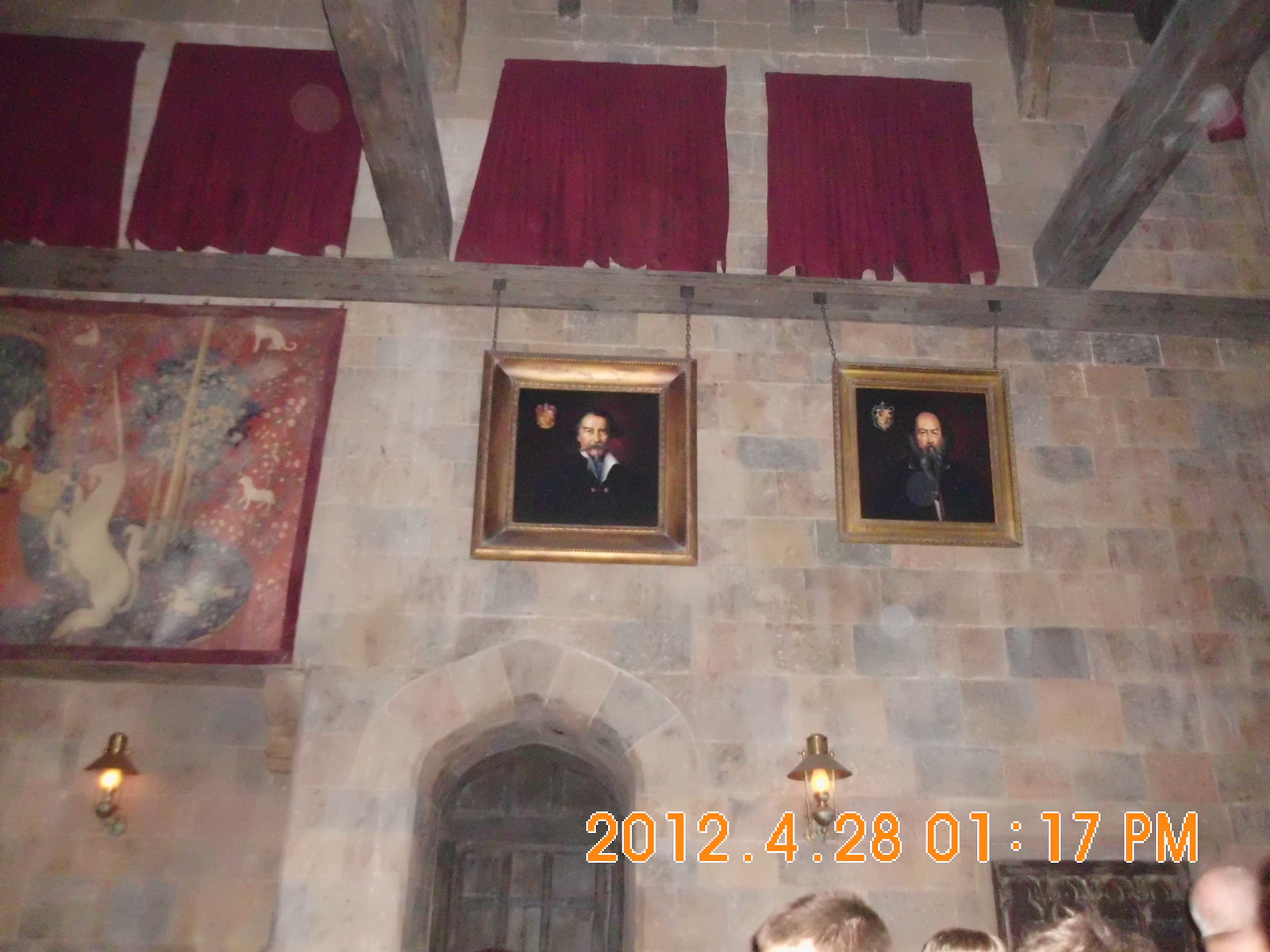The photograph captures the interior of what appears to be an ancient castle, with high, unseen ceilings and stone walls in shades of brown and beige. Central to the image, slightly left of center near the bottom, is a wooden door framed by an archway. From above, wooden rafters hang, adorned with two gold-framed portraits of stern-faced, bearded Caucasian men, each portrait embellished with a crest in the top left corner. These paintings are partially covered by maroon curtains, which appear wrinkled. Above the rafters, more portraits are concealed by red fabric. In the bottom right corner, a date and time stamp in orange font indicates the photo was taken on April 28, 2012, at 1:17 pm. Additionally, the tops of some people's heads, likely part of a tour group, are visible in the lower right area, suggesting that the room is part of a guided tour through the castle.